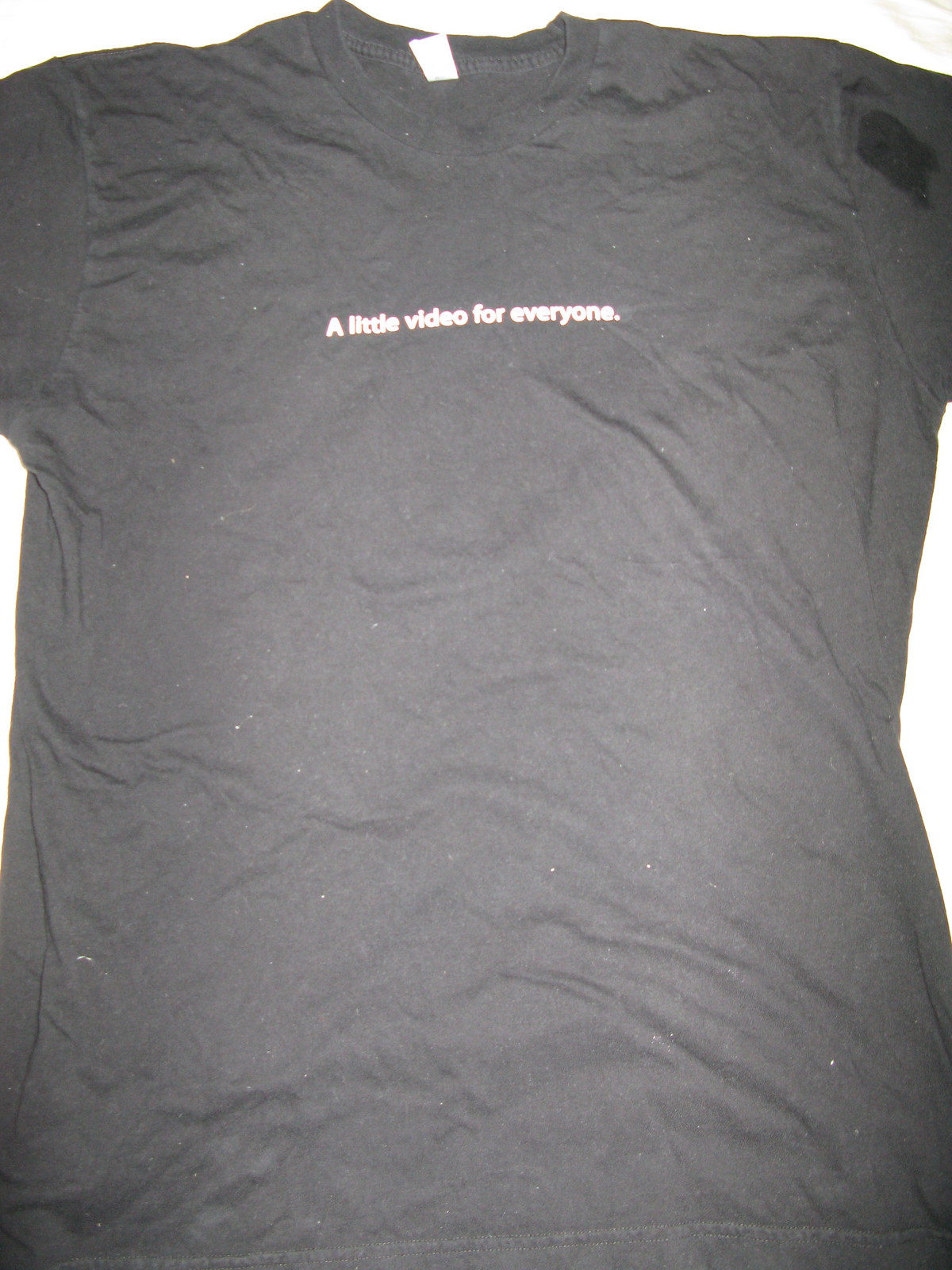A photograph captures a black, short-sleeved t-shirt centrally positioned within the frame, occupying nearly the entire image. The t-shirt is made of soft material, but appears wrinkled and is speckled with numerous small white particles that could be either dust or lint. At the neckline, a white tag is visible, bearing the inscription "a little video for everyone" in small white letters. Notably, there is a dark stain, about the size of a quarter, marring the right sleeve. The bottom hem and the sleeves are partially cropped out of the picture, focusing attention on the midsection and detailing.